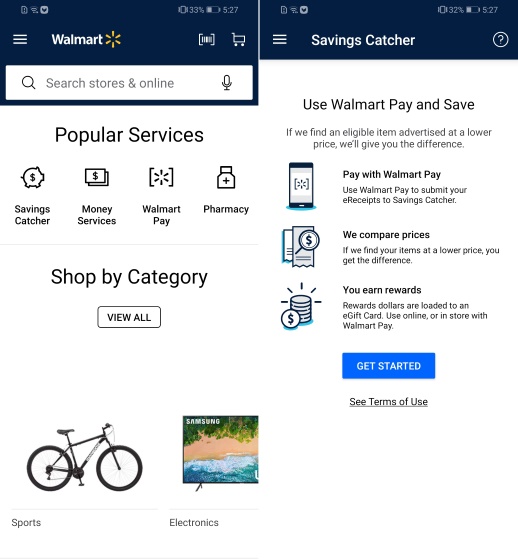This image features two side-by-side screenshots of the Walmart mobile app displayed on a smartphone. Both screenshots include typical phone status indicators: signal strength in the top left, and battery status and time (5:27 PM) in the top right. In the screenshot on the left, the battery is at 33%, while the right screenshot shows it at 32%. Additionally, both screens display a vibrate icon.

The left screenshot highlights the main interface of the Walmart app. At the top, there is a banner with the Walmart logo, accompanied by a "burger" menu icon on the left for settings, a barcode scanner icon, and a shopping cart icon on the right. Below this banner is a search bar for user inquiries. The section titled "Popular Services" follows, listing four options from left to right: Savings Catcher, Money Services, Walmart Pay, and Pharmacy. Underneath, a "Shop by Category" section is displayed with a "View All" button. Two categories are specifically shown: "Sports," featuring a bicycle icon, and "Electronics," depicted with a television icon.

The right screenshot focuses on the Savings Catcher feature. The header reads "Savings Catcher," followed by a description: "Use Walmart Pay and save. If we find an eligible item advertised at a lower price, we'll give you the difference. Pay with Walmart Pay." The section further explains how the Savings Catcher works: users pay with Walmart Pay, submit their e-receipts to Savings Catcher, and the system compares prices to find any lower prices, refunding the difference in the form of reward dollars. These rewards are loaded onto an e-gift card, which can be used online or in-store with Walmart Pay. At the bottom of this section is a prominent blue "Get Started" button.